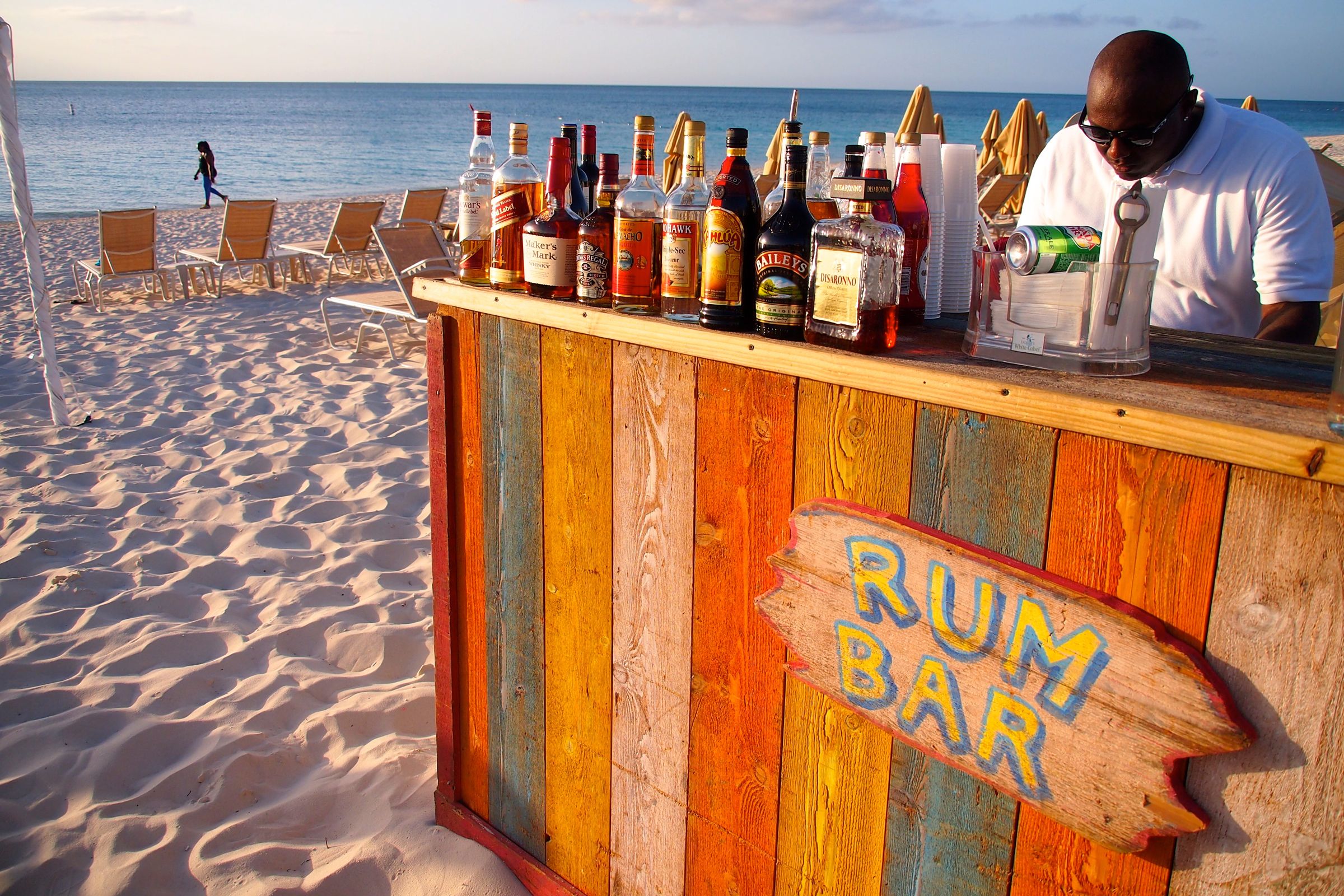In the photo, you see a vibrant scene at a beachside bar named "Rum Bar." The bar, positioned on the right side of the image, is constructed from an array of colorful wooden planks. The planks are painted in shades of blue, orange, cream, and tan, with some exposed wood panels. A piece of flattened driftwood is nailed to the front of the bar, with "Rum Bar" written in bold yellow letters outlined in blue.

Behind the bar stands an African-American bartender, dressed in a white polo shirt with the sleeves rolled up, wearing black sunglasses, and looking down at some activity he's engaged in. The bar top is cluttered with various bottles of liquor, including Maker's Mark, Kahlua, Bailey's, De Sirono, and more. There is also a plastic container holding a can of Canada Dry ginger ale, napkins, straws, and a bottle opener, alongside a stack of white plastic cups.

To the left of the bar, the scene extends to a beach with white sand. About four or five yellow beach chairs are set up on the sand, facing the ocean. A person is seen walking along the shoreline in the left-hand corner of the image. The background features a stunning view of the blue ocean, accompanied by a few yellow umbrellas and a clear sky with scattered high clouds. This picturesque setting captures the idyllic blend of a lively bar atmosphere and the serene beauty of the beachfront.